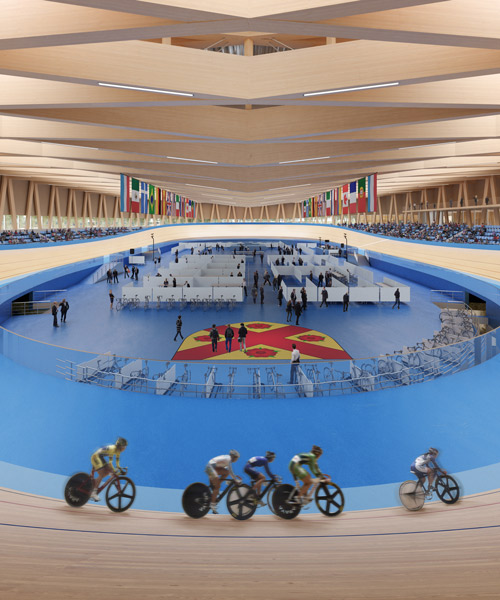The image depicts a large, circular indoor sporting venue, reminiscent of an Olympic gathering. Dominating the forefront are five cyclists on a beige track, racing towards the bottom edge of the image. Surrounding the track, the vibrant interior features a striking blue floor. In the center lies a distinct emblem featuring a red cross and a yellow shield with red circles on it. Above, the beige ceiling showcases an intricate, diamond-like pattern of cross beams. The venue offers ample seating with bleachers filled with spectators, all lining the perimeter. Numerous flags from different countries hang prominently around the venue, emphasizing its international scope. The middle area is bustling with activity; white cubicles, benches, and temporary walls host people in dress clothes, mingling and working. Bicycle racks, ramps, and other sporting equipment are scattered amidst this hive of activity, completing the dynamic scene of this high-energy athletic event.